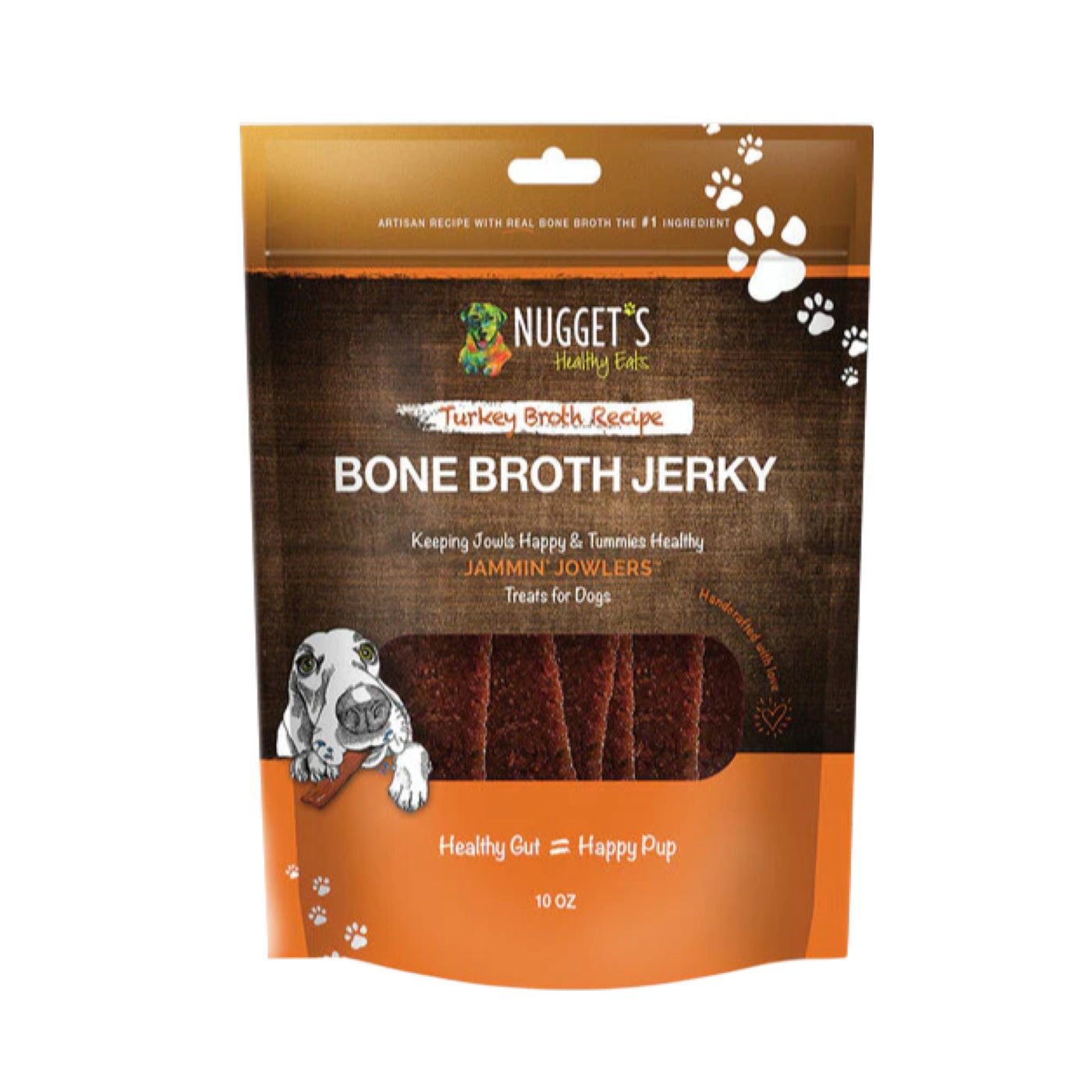The product packaging is a vertically rectangular, multi-colored print piece designed for dog treats called "Nuggets Healthy Eats, Turkey Broth Recipe, Bone Broth Jerky." Featured prominently at the top, in white text, it reads "Artisan Recipe with Real Bone Broth, the number one ingredient." The copper-colored top section includes white paw prints ascending the right side and has a hole at the top center for hanging on a rack. 

In the middle section, a window allows visibility into the bag to showcase the grainy, rectangular treats inside and is accompanied by the phrase "Keeping Jowls Happy and Tummies Healthy." To the left of the window is a black and white illustration of a dog with a large bulbous nose, paws draped over the lower brown section, making it appear as though the dog is peeking over a wall. 

The bottom portion of the packaging is orange, labeled with "Healthy Gut equals Happy Pup, 10 ounces" in white text. Additionally, the bottom left corner features small white paw prints, while larger paw prints decorate the bottom right corner, providing a playful touch. Overall, the detailed design emphasizes the high-quality, artisanal nature of the dog treats while ensuring they stand out on store shelves.